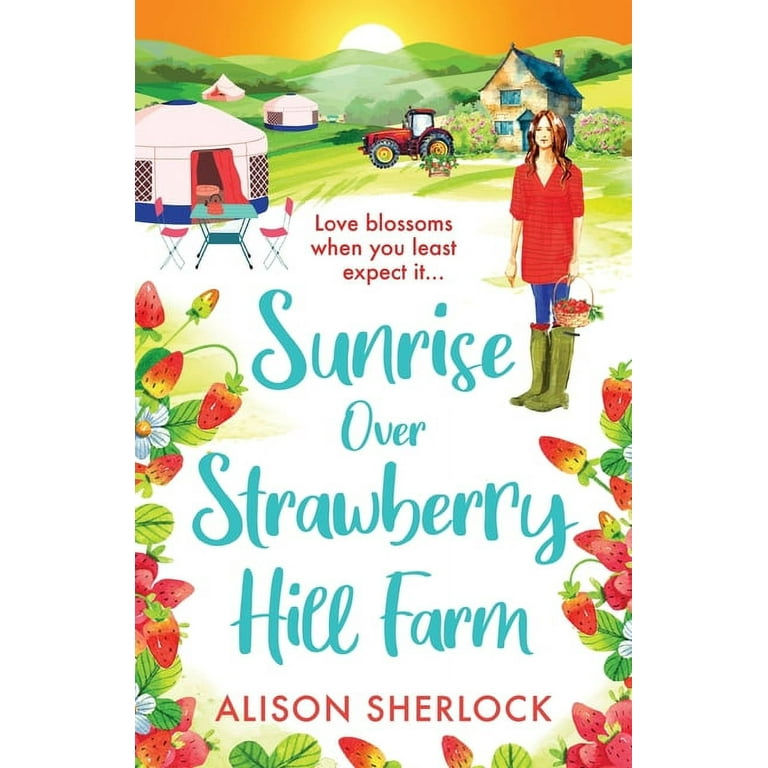The cover of the book "Sunrise Over Strawberry Hill Farm" by Alison Sherlock features a detailed, hand-drawn or watercolor-style illustration. Central to the image is a young woman with shoulder-length brown hair, dressed in a red dress, blue tights, and knee-high green waterproof boots. She holds a wicker basket filled with strawberries. The title, written in light blue text, sits prominently in the middle of the cover, just below the phrase "Love blossoms when you least expect it," which is in red text.

Surrounding the woman and the title are blooming strawberry vines. The backdrop depicts a quaint, cottage-style farmhouse, a red tractor with large back wheels, and an arrangement of tents, including a round, yurt-like structure and a triangular canvas tent. A small camping table with two red chairs and a pink kettle is set up in front of the yurt-like tent. The background showcases rolling green hills under an orange sky, indicating either sunrise or sunset. At the bottom of the cover, in simple red lettering, is the author's name, Alison Sherlock.